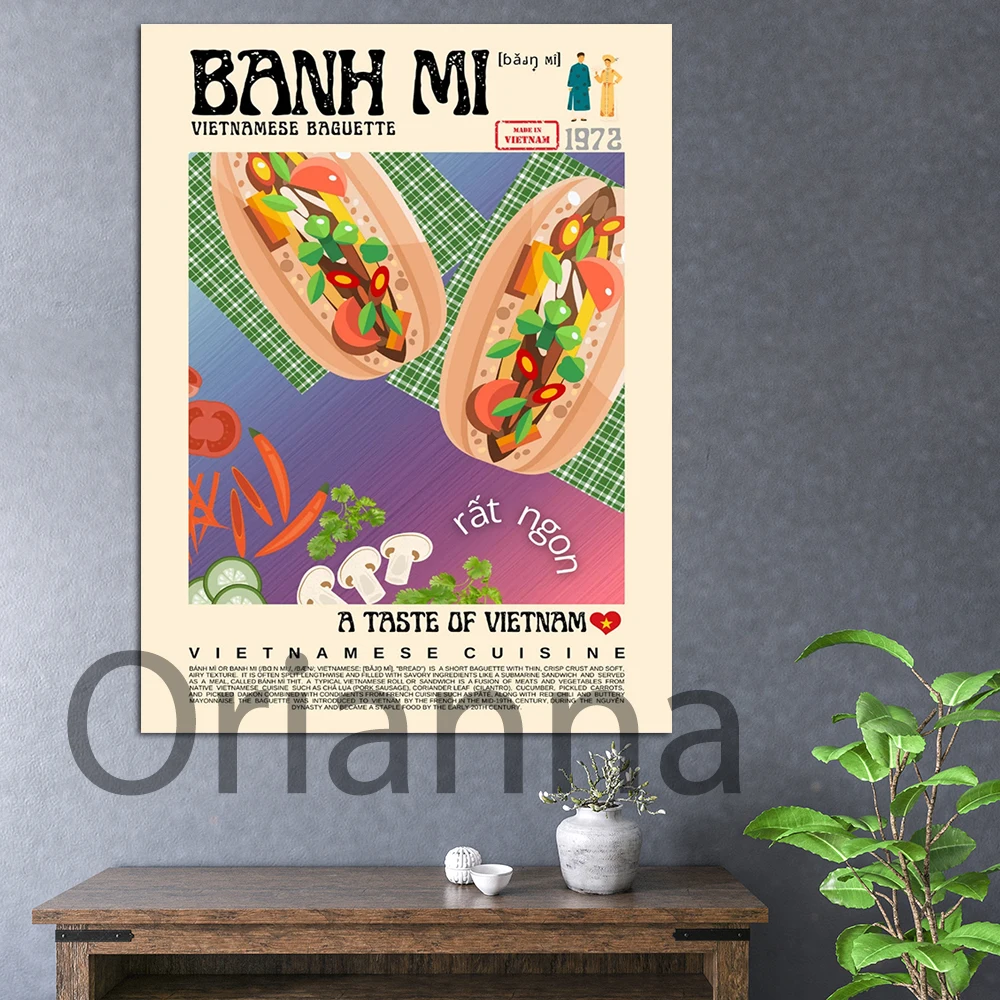Hanging on a gray wall, this poster is positioned above a medium brown wooden table. The tabletop holds a white marble vase with a plant that has white-tipped leaves, a small white cup on a saucer without a handle, and a small white trinket of comparable size. The poster itself has a creamy beige background with bold black letters at the top spelling "Banh Mi," and just below in smaller black text, it reads "Vietnamese Baguette." Prominently featured in the center is an image of two Banh Mi sandwiches resting on green plaid fabric. In the bottom left corner of the photo on the poster, there are sliced tomatoes, cucumbers, mushrooms, parsley, and carrots. Below the photograph, "A Taste of Vietnam" is written, accented with a small red heart. At the very bottom of the poster, spaced out black letters state "Vietnamese Cuisine." The entire photo on the poster has a watermark with the name "Oriana" in large black letters. On the right side of the photograph, a green floor plant is visible, adding a touch of natural color to the scene.